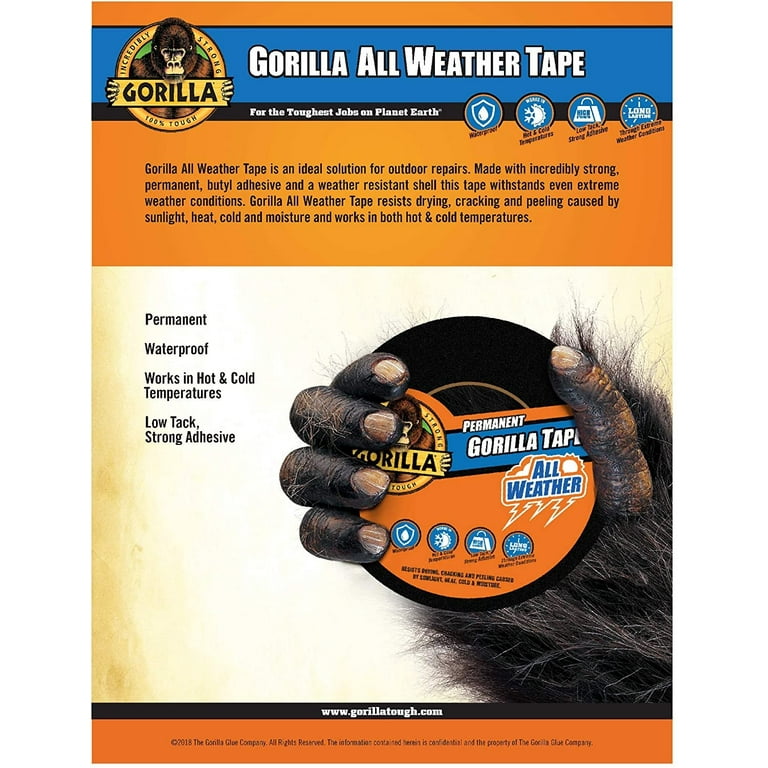This detailed image is a photograph of an advertisement for Gorilla All-Weather Tape. At the top, there is a blue band with the product's name, "Gorilla All-Weather Tape," written in bold white letters. Framing the top of the advertisement is an orange border, while additional smaller orange borders appear above and below the product name.

To the left of the title, there is a distinctive logo featuring a tough, muscular gorilla encircled by a yellow ring. The logo bears the text "Incredibly Strong, 100% Tough," with the gorilla gripping a sign that reads "Gorilla." Below this, there is an informative orange section describing the product: "Gorilla All-Weather Tape is an ideal solution for outdoor repairs. Made with incredibly strong permanent butyl adhesive and a weather-resistant shell, this tape withstands even extreme weather conditions. It resists drying, cracking, and peeling caused by sunlight, heat, cold, and moisture, operating efficiently in both hot and cold temperatures."

Beneath this informative text, the advertisement features a prominent image of a gorilla's hand holding a roll of Gorilla tape that can be purchased in stores. Adjacent to the image, there's a list of the product's key features: "Permanent, waterproof, works in hot and cold temperatures, low tack, strong adhesive." At the bottom, a black border contains the website address "www.gorillatuff.com," followed by an orange block with indistinguishable text. This visually striking advertisement emphasizes the durability and weather resistance of Gorilla All-Weather Tape, reinforcing its suitability for the toughest jobs on planet Earth.